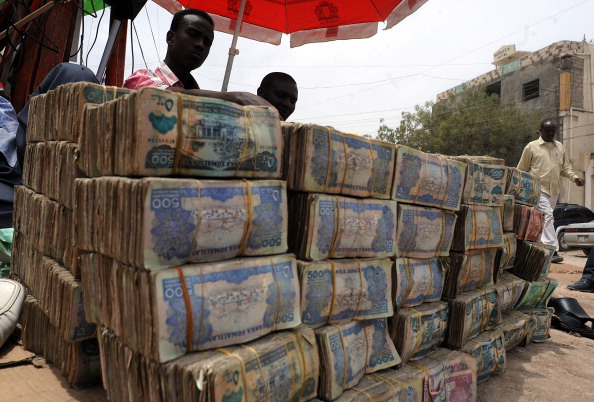In this outdoor image, an impressive display of stacked bundles of paper money dominates the foreground, each bundle meticulously tied with two orange strings. These bundles are arranged in numerous rows and columns, creating a towering formation that almost seems to engulf the scene. The stacks rest upon a ground covered with sand, evoking a street market atmosphere, possibly in a third-world country.

Behind this colossal arrangement of money, two dark-skinned men stand out. The man on the left sports a red and white shirt while his companion on the far right wears a striking yellow long-sleeved button-up shirt paired with white pants. Above them, providing shade, is a red and white umbrella held up by a white pole.

In the background, to the far right, a third dark-skinned man is seen walking past a multi-story building with gray concrete siding. A patch of greenery from a tree enhances the background. The sky is clear, revealing no signs or text to distract from the scene's rich details. The diverse palette of colors within the image includes shades of dark red, gray, blue, green, pink, and yellow, adding vibrancy to the captured moment.